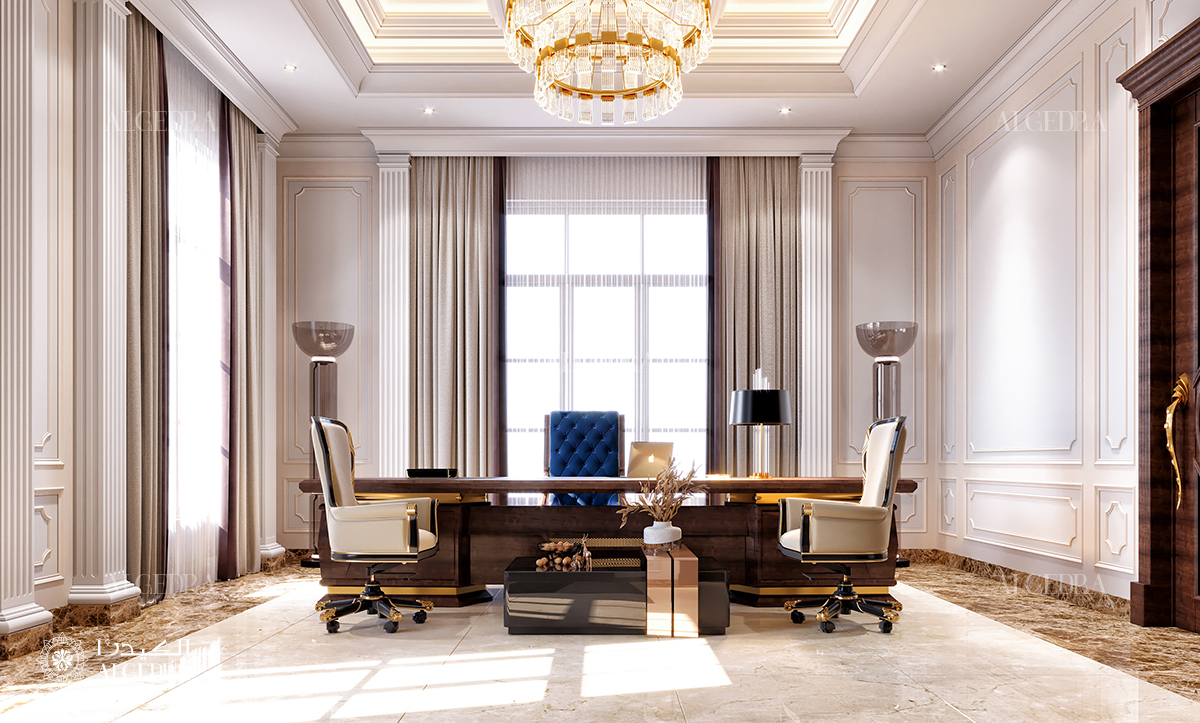This photograph captures the opulent interior of a luxurious, well-appointed room. Dominated by tall ceilings, the space exudes elegance with its glossy beige marble floors adorned with a border of rich brown marble. The walls are predominantly white, featuring ornate framed sections running along their surfaces.

At the center of the back wall, a large rectangular window flanked by beige curtains invites an abundance of natural light. The ceiling, also white, is graced by a stunning circular glass and gold crystal chandelier, drawing the eye upward.

In the middle of the room stands an imposing brown wooden desk, accompanied by a blue velvet tufted chair behind it and two stylish office chairs in front. The chairs in front have ivory upholstery with black legs and gold accents, redefining opulence. On the right side of the table, there is a black lampshade. The desk itself holds an open MacBook, showcasing the familiar Apple logo.

A wooden door with a golden handle is partially visible on the right wall, adding a touch of classic sophistication to the room's overall grandeur.